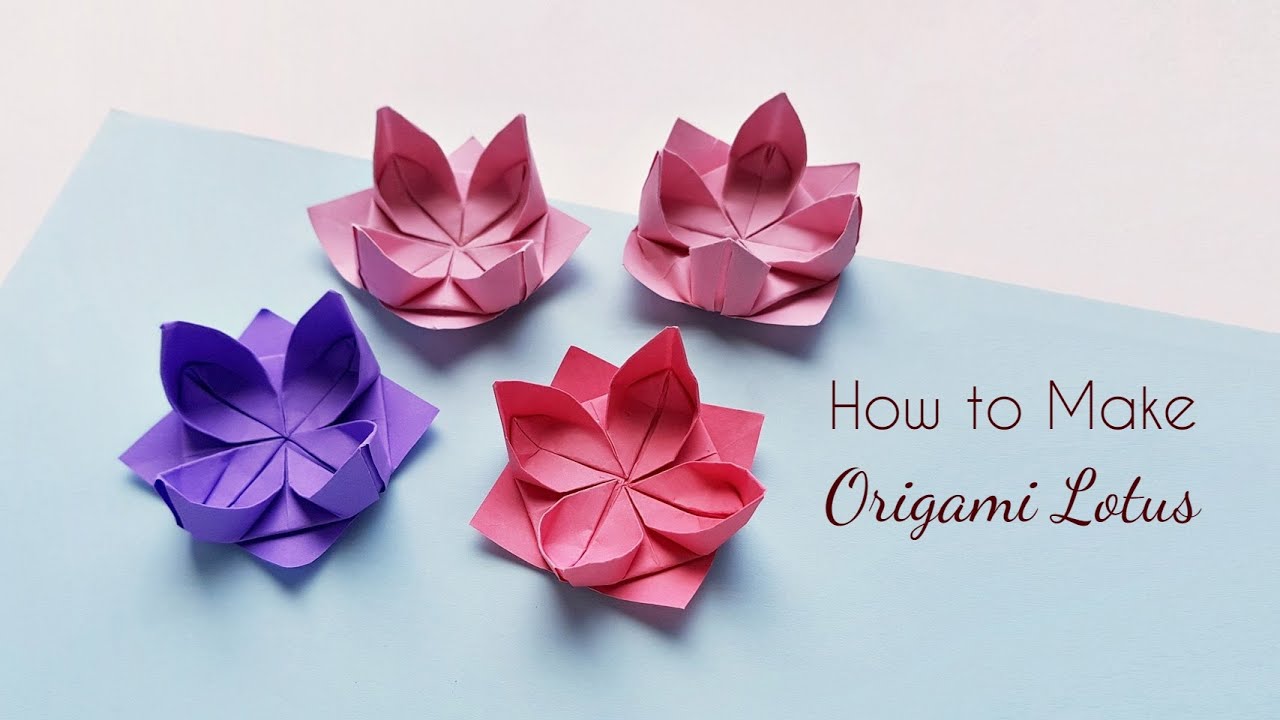The image is a color photograph featuring a pinkish background with a light blue piece of paper sitting on the table. Prominently displayed are four origami flowers: two deep pink blossoms at the top, and on the bottom, one purple flower to the left and a bright pink flower to the right. These flowers are lit from the back, casting shadows toward the camera. On the right side of the image, the text "How to Make" is printed in a regular font, and below it, "Origami Lotus" is written in cursive, both in a brown or burgundy color. The careful arrangement and delicate lighting highlight the detailed craftsmanship of the multicolored origami lotuses.